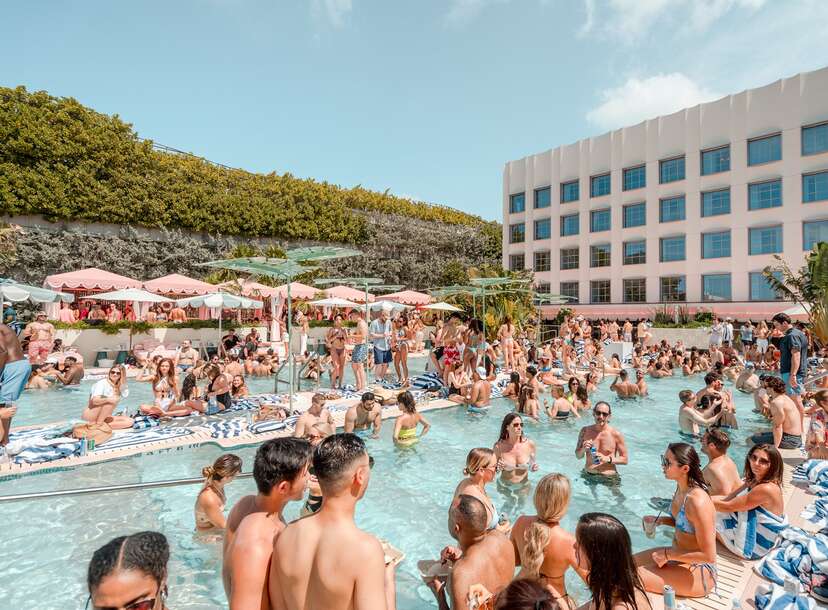The image captures a bustling outdoor pool scene, teeming with at least a hundred young people, mostly in their 20s or late teens, dressed in swimming attire. The pool, about three to four feet deep, is packed with people standing and chatting casually. In one section of the pool, a floating catwalk or center walkway area features numerous green umbrellas, providing shade for those lounging around. Others are seated along the pool’s edge, particularly in the lower right corner of the photo, draped in blue and white striped towels.

A striking swim-up bar serves as a central social hub within the pool. Surrounding the pool on the deck are additional green and white umbrellas, while further out, an array of peach-colored umbrellas offers more gathering spots. Behind the vibrant pool scene stands a five-story building with a white cream facade and numerous blue-tinted glass windows arranged in a grid pattern. This structure exudes a modern, hotel-like appearance.

Beyond the pool's retaining wall, adorned with rough foliage such as juniper bushes, a slightly elevated area features bar or tent-like structures for further leisure activities. The background displays a lush hill with greenish-brown vegetation under a partly cloudy, light blue sky, adding an inviting natural element to the lively atmosphere.